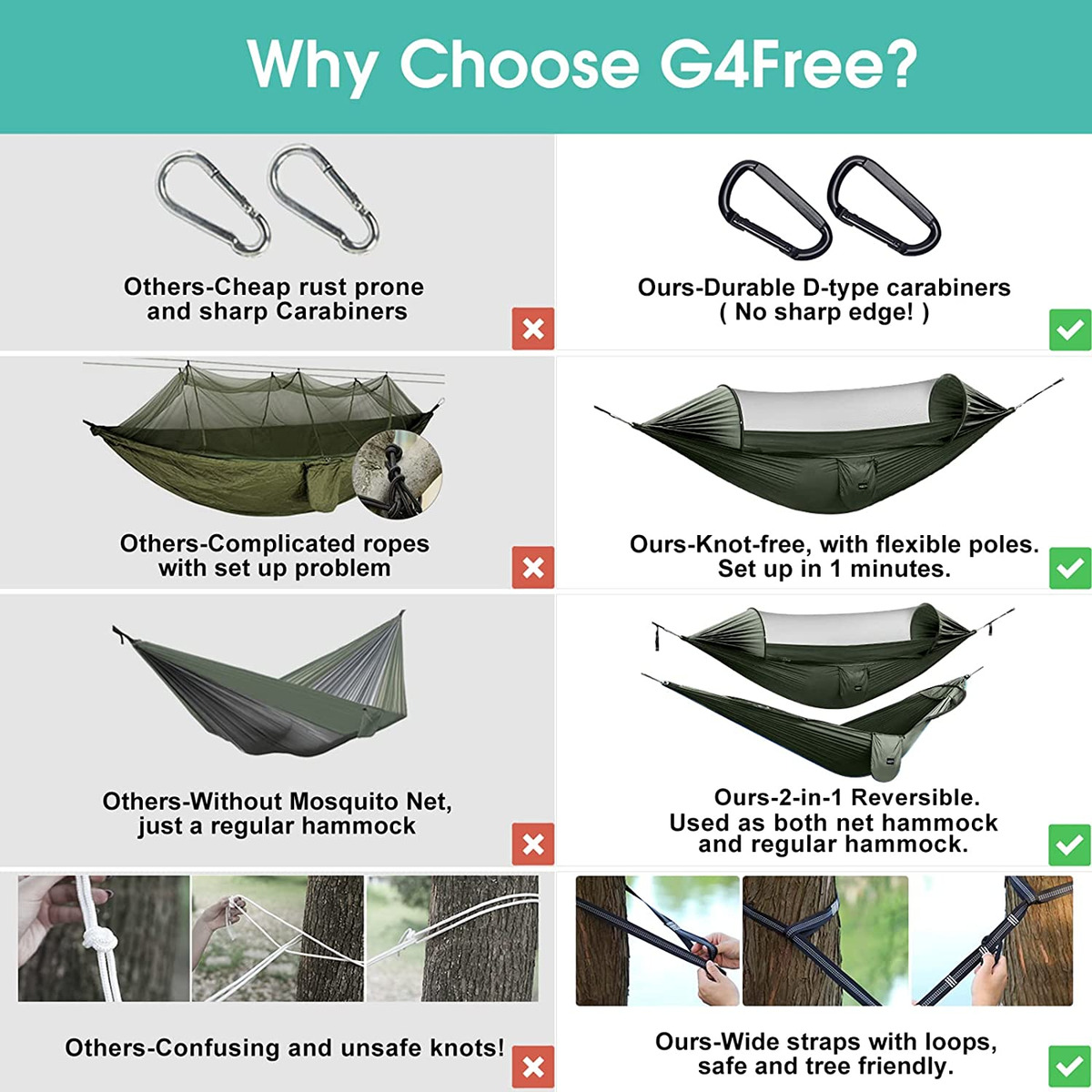This detailed and comprehensive caption describes a photograph showcasing various camping gear items available for sale at a dedicated camping store. The promotional material is titled "Why Choose G4Free" with the text prominently displayed across the top. The featured products include essential camping tools such as carabiner clips, ropes, hammock setups, and mosquito net-covered hammocks. It also provides practical illustrations on how to securely tie knots for setting up hammocks between trees, emphasizing safety and ease of use. The advertisement highlights the benefits of using specialized straps over traditional knots for enhanced security and convenience. The carabiners shown are the type commonly used by climbers, ensuring reliability and strength.

Visually, the ad is organized into a grid layout comprising a total of 14 images: four rows with two images each, along with a bottom row containing six images, resulting in a balanced, square-shaped visual format suited for placement in magazines or newspapers.